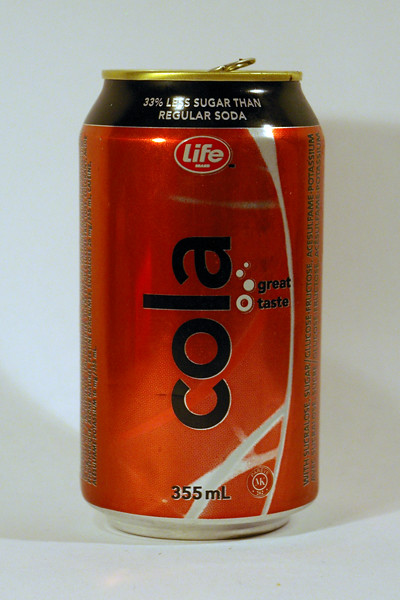The photograph captures a soda can on a white surface with a white background. The can prominently features a red body with a gold top and silver bottom. A distinct black band encircles the top of the can, which is adorned with the text "33% less sugar than regular soda" in bold lettering. On the red portion, there is a circle with a white outline and red interior, marked with the brand name "Life." Below the circle, the word "Cola" is displayed prominently, paired with the phrase "Great Taste." The can also bears the volume "355 milliliters" at the bottom. Faint readable details include ingredients like sucralose, sugar/glucose-fructose, and acesulfame potassium printed along the side, accompanied by reflections and a stamp with "NK" at the bottom right. This image is somewhat dimly lit, emphasizing the rich color and metallic sheen of the can.